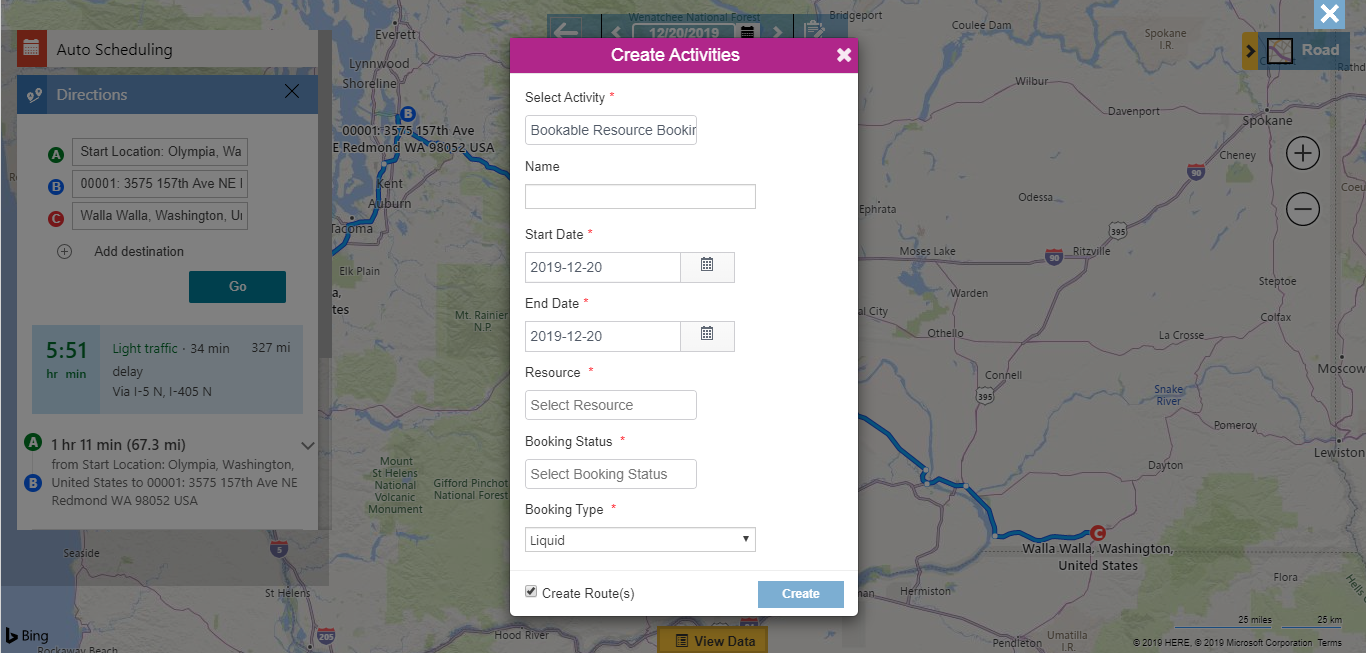The image depicts a detailed interface of a map-based website or web application. The primary focus is a pop-up window centered on the screen labeled "Create Activities." This window prompts the user to input relevant information such as activity name, start date, end date, resource, booking status, and booking type.

In the background, a map of Washington State is visible, highlighted with a marked trail or destination. Prominent city names such as Bold and Walla Walla indicate that the map is indeed focused on this region. Another window to the left shows the user's planned route, including starting and ending points, providing a comprehensive overview of the travel or activity planning process offered by the website.